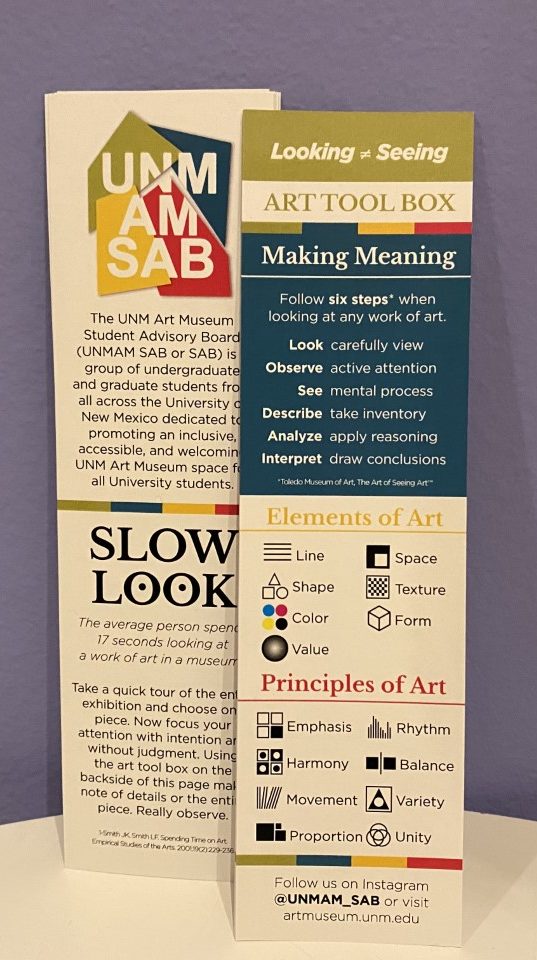This photograph captures two prominently displayed posters set against a purple-colored wall. The posters belong to the University of New Mexico Art Museum Student Advisory Board (UNM AMSAB), an inclusive and welcoming group of undergraduate and graduate students dedicated to promoting art accessibility at the university. 

The left poster, with a white background and predominantly black text, provides insights into navigating an art exhibition. It encourages viewers to engage deeply with artwork by following six steps: looking carefully, viewing, observing with active attention, seeing as a mental process, describing and taking inventory, analyzing with reasoning, and interpreting to draw conclusions. This methodology is referred to as the "Art Toolbox."

The right poster, characterized by a light green, white, dark blue, and cream-colored background, elaborates on the foundational elements and principles of art. It emphasizes that "looking is not equal to seeing" and outlines key art elements such as line, shape, color, value, texture, and form. It also lists the principles of art, which include emphasis, harmony, movement, proportion, unity, variety, balance, and rhythm. Additionally, it provides the group's Instagram handle for further engagement.

Together, these posters not only guide museum visitors on how to thoughtfully engage with art but also highlight the values and contact information of the UNM AMSAB.